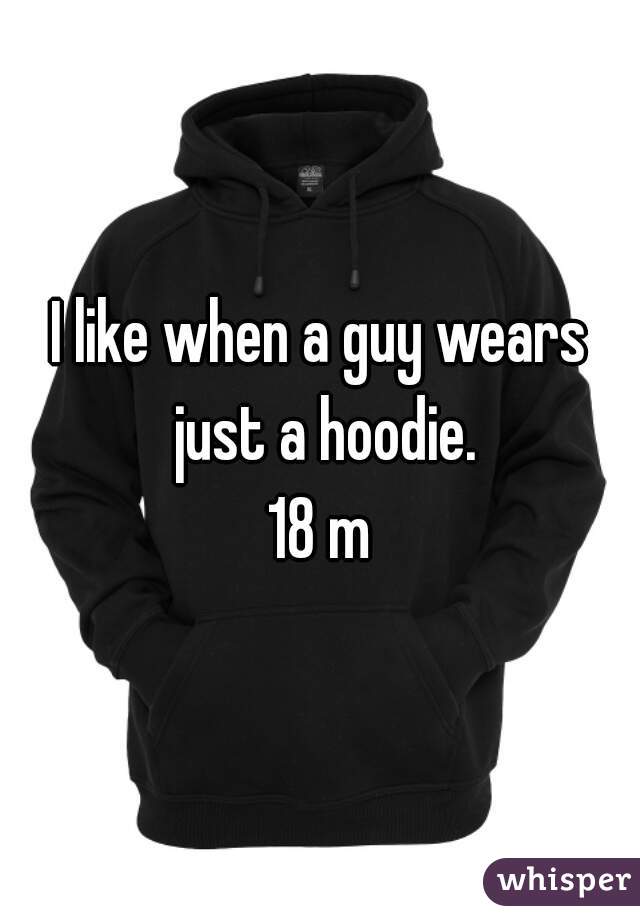The image is a meme featuring a plain black hooded sweatshirt against a white background. The hoodie appears to be filled out as if on a mannequin, with the cuffs tucked into the front pouch pocket. The fabric has drawstrings, and a tag is faintly visible inside the hood. Superimposed in white text across the hoodie, it reads, "I like when a guy wears just a hoodie." Below this, the notation "18M" is displayed. In the bottom right corner, the word "whisper" is written in lowercase white text within a purple, rectangular button-shaped border. The overall quality of the image is somewhat low-resolution and slightly blurry, with no visible shadowing, giving it a simple and straightforward appearance.